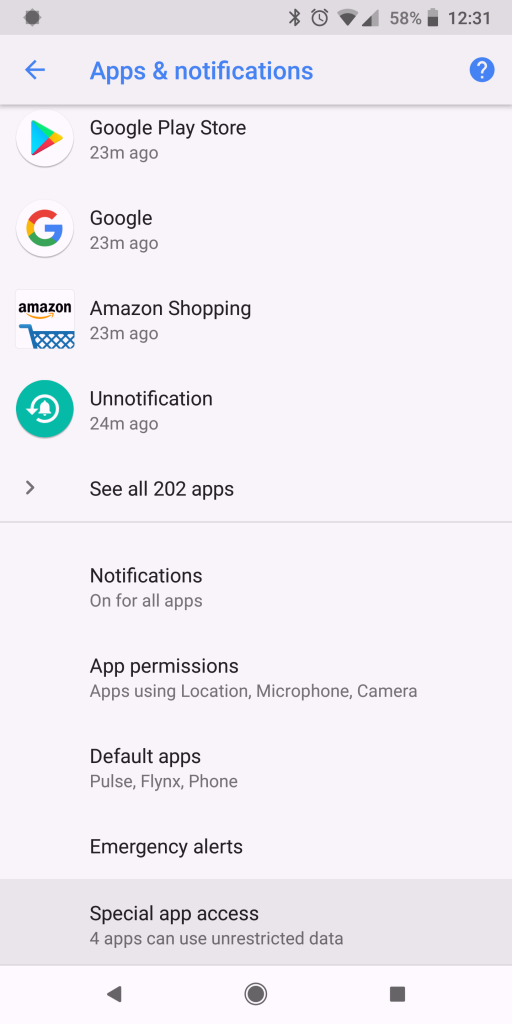The screenshot captures a smartphone's "Apps & Notifications" menu as displayed at 12:31 PM, with various status indicators at the top. These include an active alarm, enabled Bluetooth, cellular signal strength, and a battery level at 58%. The top bar features a navigational back button and a blue question mark icon.

The primary section of the screenshot shows a list of recent activities for apps. At the top, the Google Play Store, marked by its colorful triangle logo in blue, green, pink, and yellow, is noted as used 23 minutes ago. Similarly, the Google app, identifiable by its multicolored 'G' logo, is reported as accessed 23 minutes ago. Amazon Shopping, with its signature smiling cart logo, also shows activity 23 minutes ago. An unnamed notification appears 24 minutes ago, represented by a teal alarm clock icon encircled by a white arrow.

Further down, there are detailed settings options:
- Notifications: Setting for all notifications, including options to turn them on for all apps.
- App Permissions: Information on which apps are using the location, microphone, and camera.
- Default Apps: Including settings for SMS (Pulse), browser (Flinks), and phone.
- Emergency Alerts: Configurations for receiving urgent notifications.

At the bottom, "Special App Access" lists apps that can utilize unrestricted data.